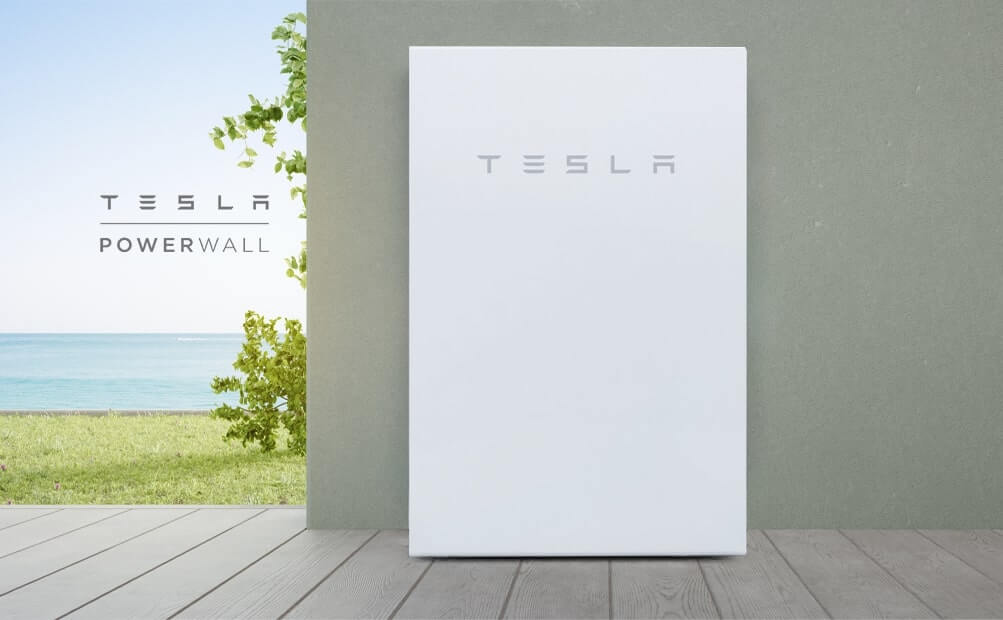The image showcases a detailed setting possibly on a deck. The bottom part prominently features wooden planks that extend across a substantial portion of the frame. At the center of the deck is a large white block, dominating the photo's middle section. The white block has the word "Tesla" centered towards the top in gray font. Behind the white block, a half wall extends from the right edge of the image but stops shortly after reaching the center, continuing upwards until it goes out of the frame. The scene gives a structured and minimalist feel, highlighting the central white block with the Tesla branding against the wooden deck backdrop.